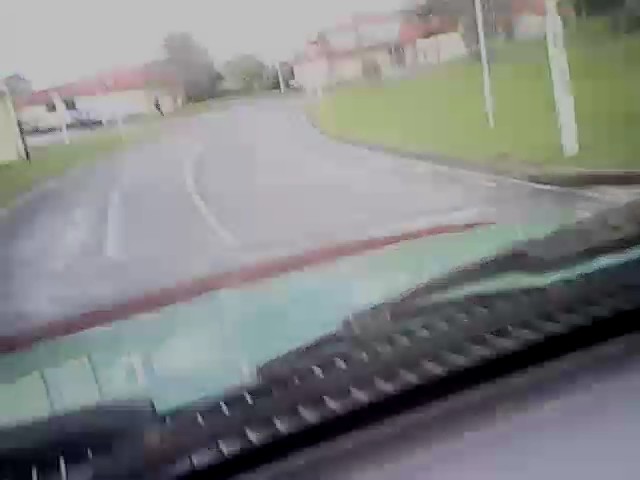A highly blurry dash cam photo taken from the front seat of a car shows the dashboard, windshield wipers, and a green-hooded vehicle driving down a gray, wet residential street on a rainy and cloudy day. The surroundings include green grass and greenery on both sides, with embankments around the edges and poles flanking the sides of the road. In the distance, two tan houses with red roofs are visible on either side of the street. The road itself is lined with faint white lane markings, and the overall scene appears to be part of a cohesive community due to the similarity in the buildings' design and close proximity. Tall, leafy trees rise into the gray sky, adding to the overcast atmosphere. Despite the poor image quality, faint details like the car's interior vent along the window and the lack of other traffic can be discerned, hinting at a quiet residential area.